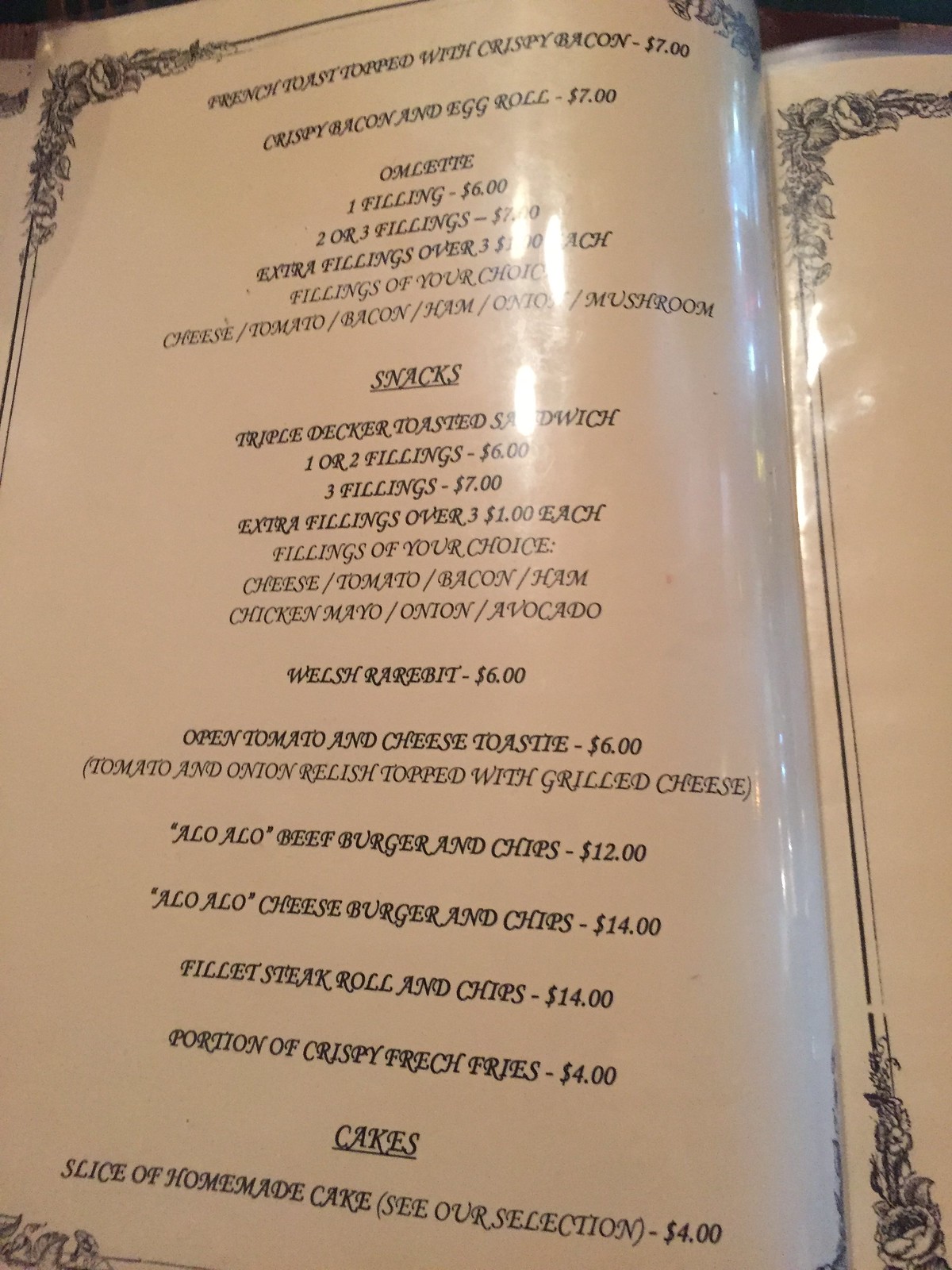An open book displays a detailed, laminated menu. The left page occupies about three-quarters of the visible area, while the right page extends off-screen, curving down with about an inch of its border visible. Elegant floral designs adorn the borders of the pages, prominently appearing in the top right corner on the left page.

At the top of the menu on the left page, today's special is highlighted: "French Toast topped with Crispy Bacon" priced at $7. To the right of this item, in black lettering, it lists "Crispy Bacon and Egg Roll, $7." Further down, an "Omelet" section features various fillings with corresponding prices on the right.

The menu continues with a "Snacks" section, underlined and comprising approximately ten snack options with their respective prices listed beside them. At the bottom, the "Cakes" section is also underlined, featuring a singular item: "Slice of Homemade Cake. See our selection, $4."

Overall, the presentation of the menu is organized and visually appealing, with clear categorization and artistic flourishes enhancing its elegance.